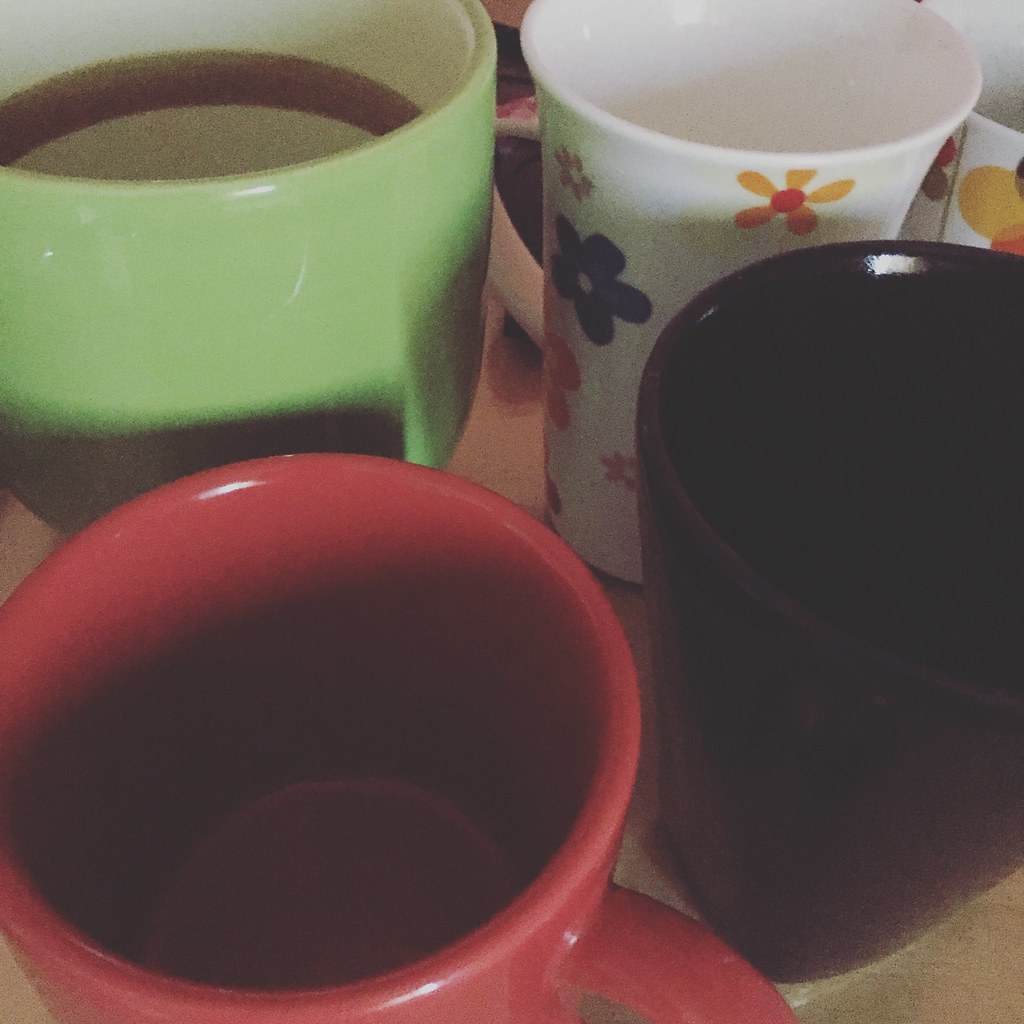This image, captured from a slightly diagonal top-down perspective, features four different cups arranged in a roughly square formation, taking up the entire frame. Starting from the upper left, there is a light green mug with no visible handle, its interior marked by a prominent brown coffee stain about halfway up. To the upper right, there's a narrow white paper cup adorned with a variety of colorful flower designs including yellow, purple, pink, and other partial blooms that extend around its curve; the cup appears empty or contains an inconspicuous liquid. Moving to the lower left, a red ceramic coffee cup, paired with a matching red saucer and visible from its base, appears empty with a slight shadow cast over its interior. Finally, to the lower right, there's a dark eggplant-colored mug, almost black, which is slightly wider than the floral cup above it, and a faint light reflection is visible on its rim, suggesting it is empty.